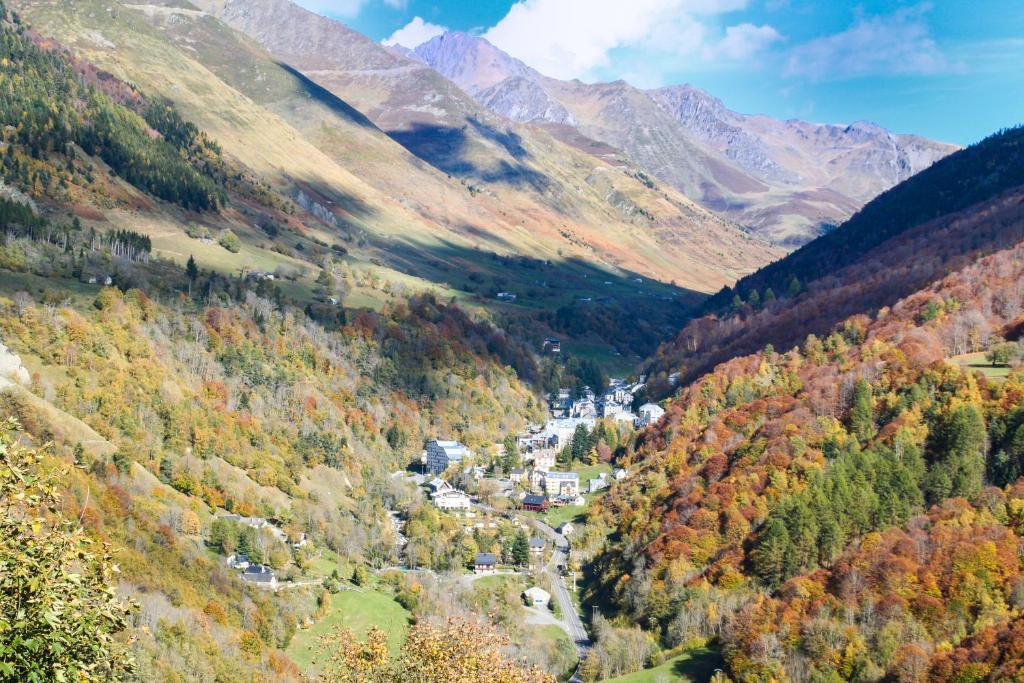The image is a horizontal rectangular scene depicting a mountain valley with several large mountains on either side, their peaks extending beyond the frame. The valley hosts a cluster of mostly white buildings, suggesting a small town or village, complete with visible streets and power lines running through the landscape. The buildings vary in size, hinting at both large beautiful homes and smaller cabins, forming a tight-knit community. The mountains on the left are adorned with trees exhibiting vibrant fall colors in shades of orange, gold, and green, contrasting with rocky cliffs visible elsewhere. In the far background, the largest mountain appears light gray, gradually darkening to brown as it approaches the foreground. The scene features an open field area to the left and patches of grass on the right, with the bottom of the image revealing more detailed natural elements like grassy weeds and bushes. Partially obscured by clouds, shadows cover the far end of the village, while the upper right corner provides a glimpse of clear blue sky.